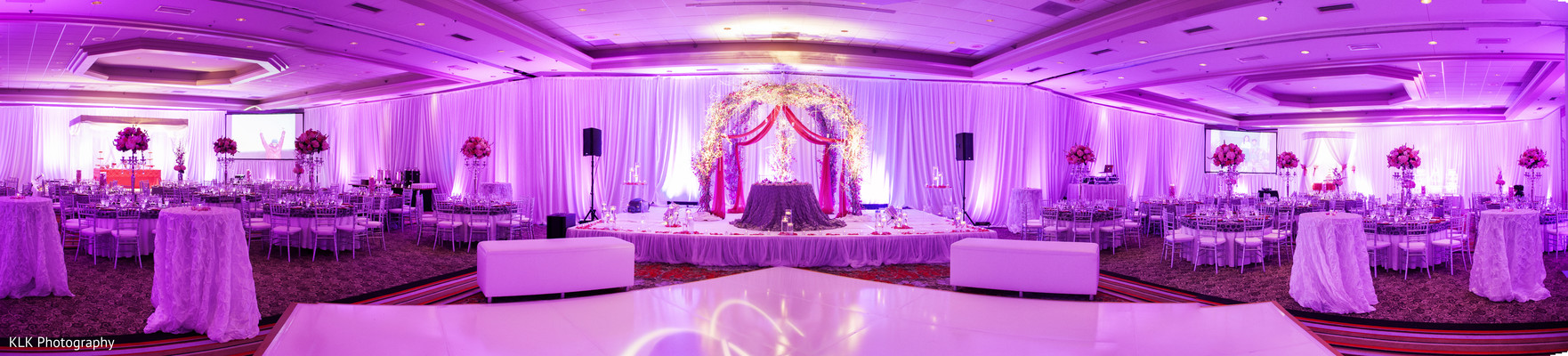This panoramic image captures a vibrant wedding reception hall with subtle details adding to its grandeur. The entire scene is bathed in a luminous pink-purple light, giving the white decor a magical hue. In the bottom left-hand corner, "KLK Photography" is inscribed in white print. The symmetrical arrangement features numerous tables draped in long, lacy tablecloths and surrounded by chairs, all glowing under the tinted lighting. Central to the room is a stage, adorned with a gold archway and cascading ribbons in red and purple hues, presumably for the bride and groom's seating. Flanking the stage are speakers, while behind it, a curtained wall adds elegance. The tables are set with tall, pink floral centerpieces that stand out against the soft brown carpet. The room's ambiance is further enhanced by various lights accenting the walls and fairy lights intertwined with draped fabrics, creating a cozy and inviting atmosphere.